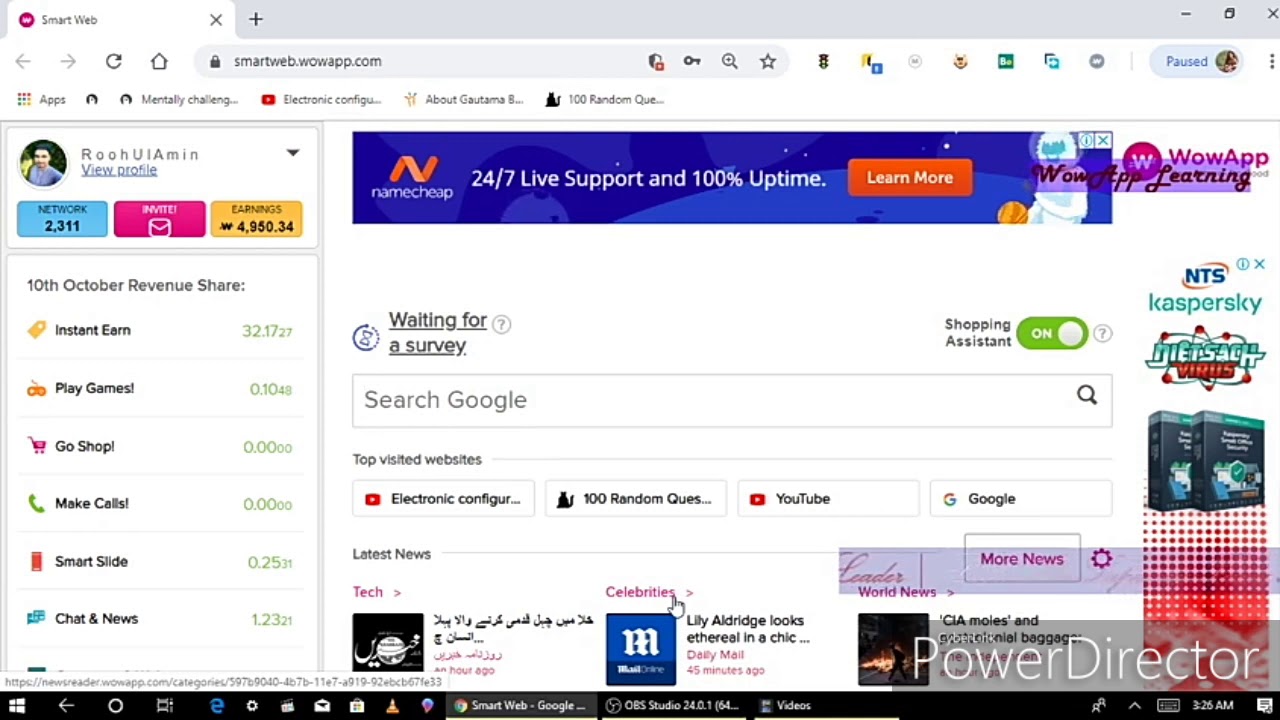This vibrant and colorful website, titled "SmartWeb," showcases a dynamic and user-friendly interface. Located in the upper left-hand corner, a striking purple and pink circle draws attention. A sleek gray search bar, labeled "smartweb.wowapp.com," spans the top, providing easy navigation.

Central to the page is Ru Yimin’s profile, which can be accessed by clicking on his name in blue text. The main section of the website features a blue background with bold text that ensures important information stands out. Prominently displayed are phrases like "24/7 life support" and "100% uptime," emphasizing the reliability of the service. An inviting orange box labeled "Learn More" beckons users to explore further.

To the left, under the "Wow App" banner, a notice states "waiting for a survey," followed by a "Search Google" bar and a "Shopping Assistant" toggle indicating it is active. Below, "Top Visited Websites" lists popular links such as "electronic configuration," "100 random something," "YouTube," and "Google."

The left sidebar highlights "The Network 2311," with a prominent pink "Invite" prompt and earnings of "4950.34." The text also mentions the "10th October revenue share." The sidebar continues with options like "Instant Earn," "Play Games," "Go Shop," "Smart Slide Chat," and "News," providing a variety of interactive features for the user.

In the lower right-hand corner, the term "Power Director" is prominently displayed, rounding off the comprehensive overview of the site's offerings.